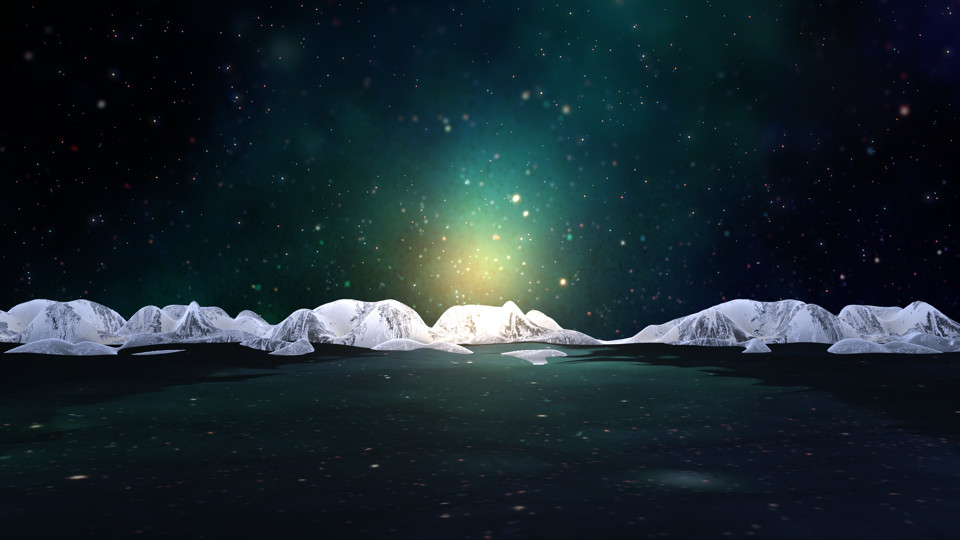The image depicts an ethereal nighttime scene where the sky is adorned with a vast array of stars and a subtly shining moon, creating a dark, cosmic ambiance. Across the center and spreading slightly toward the bottom are six striking white icebergs, laid out on an expansively flat, glossy body of water. The water reflects the dark sky intermixed with colors like yellow, red, and blue, which appear as tiny specks of light. These reflective hues add a dreamlike quality to the photograph. The sky exhibits a gradient of dark blue and green, with hints of light yellow suggesting a distant fiery sun setting, casting a mystical glow over the scene. On the far right, a black structure and a planetary body hover, contributing to the celestial atmosphere of the artwork. The icebergs, resembling snow-covered mountain ranges or possibly tents without openings, are tightly clustered, enhancing the serene, otherworldly feel of the image.